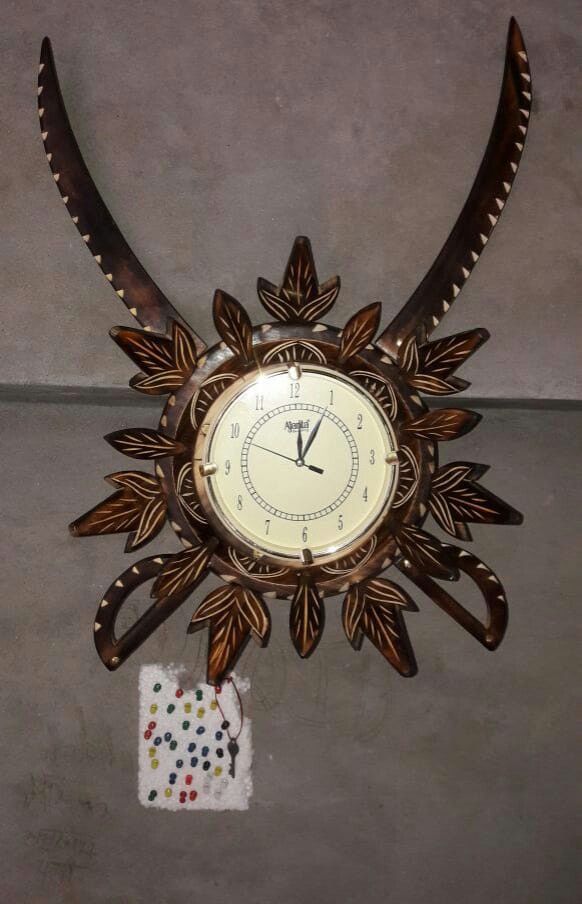A photograph showcases a highly ornate clock mounted on a two-tone, vertically divided wall. The lower portion of the wall is painted in a richer, darker gray, while the upper section contrasts with a lighter gray shade. The clock face features a golden pale yellow hue, with classic black minute and hour hands, complemented by a black second hand. The time displayed on the clock is 12:05. Encircling the clock's face are the numbers 1 through 12, and directly beneath the '12' is an illegible brand name. A circular ring outlines the clock's numerals, adding another layer of detail. The clock is framed by an intricately carved wooden border, artistically shaped into an elaborate leaf pattern that extends outward from the clock face. Two prominent, blade-like extensions protrude from the top, enhancing the clock's dramatic and ornamental appearance. The wooden carvings are primarily brown with subtle yellow highlights, adding depth and richness to the textured design.